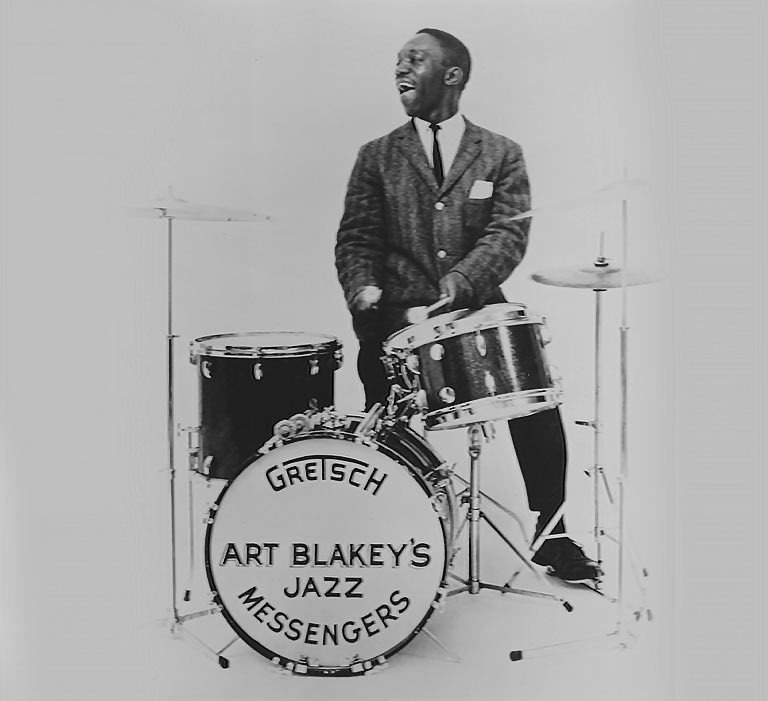This detailed black and white photograph captures an African-American man, likely from the 1940s or 1950s, seated behind an elaborate drum set, exuding joy as he appears to be smiling or possibly singing while playing the drums. The drum set features a large floor drum with "Gretsch" written at the top and "Art Blakey's Jazz Messengers" emblazoned on the bottom, indicating the band’s name. There are three smaller drums on stands and two symbols on stands—one on the left and a slightly lower one on the right. The man is immaculately dressed in a gray striped suit, a white shirt, a black skinny tie, and black shoes. The suit jacket is buttoned up and adorned with a white handkerchief in the pocket. The simple white background of the photograph further highlights the drummer's engrossed performance, showcasing the era's quintessential jazz scene.